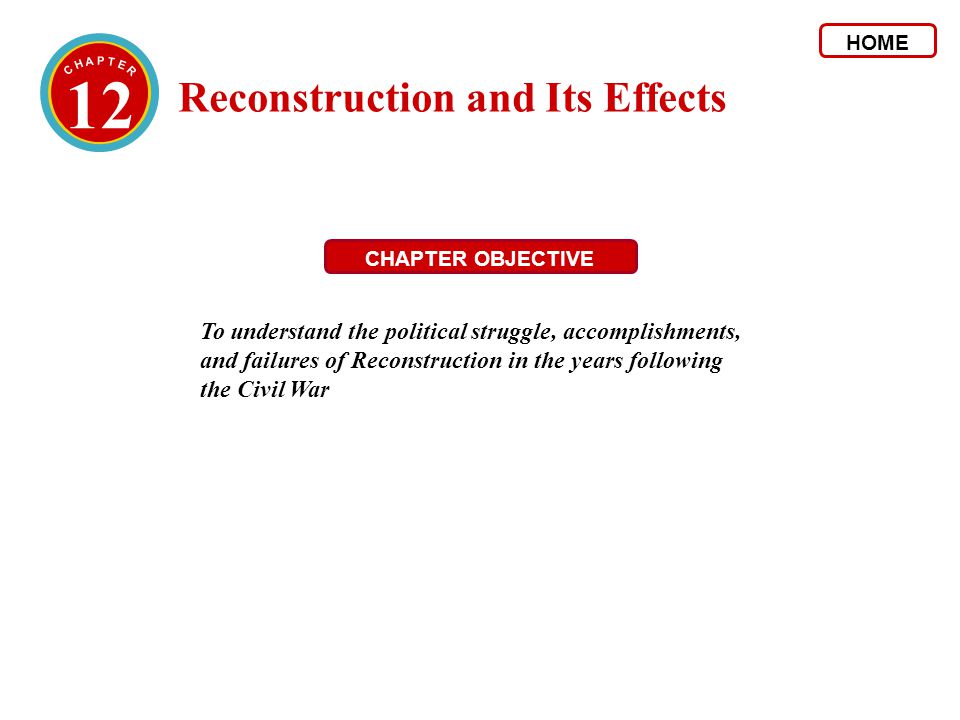The image features a page with a white background prominently displaying red and black text. In the upper left corner, there is a circle outlined with thin blue and yellow circles, containing the text "Chapter 12" in white print. To the right of the circle, the main title "Reconstruction and its Effects" is written in bold red lettering. On the upper right, a black text "Home" is enclosed in a red rectangle. Centrally positioned below the title is another red rectangle with the white text "Chapter Objective." Below this, in black print, is the objective statement: "To understand the political struggle, accomplishments, and failures of Reconstruction in the years following the Civil War." The overall style suggests it is a page from an educational book or a website slide, with the structured layout and informative content reinforcing this purpose.